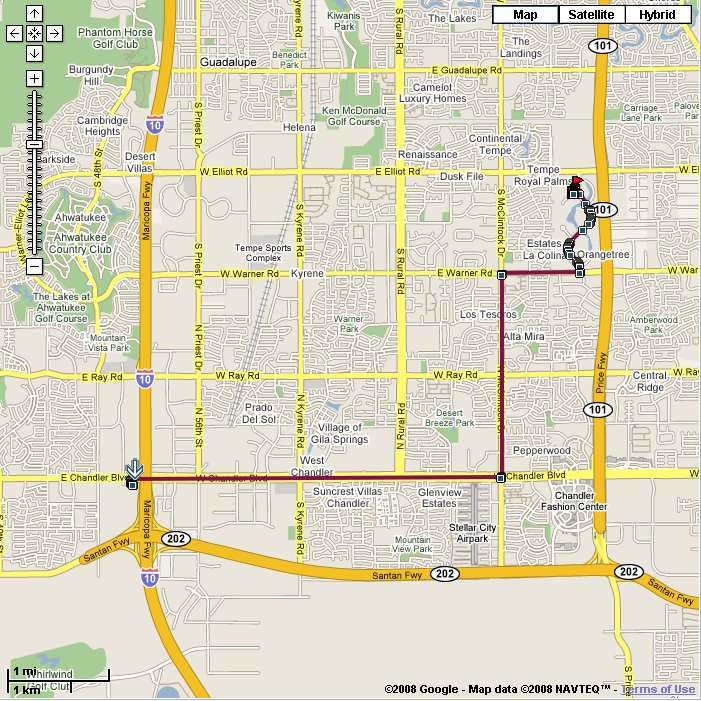The image depicts a detailed map, potentially sourced from MapQuest or Google Maps. This map covers an area with multiple highways and main streets. Prominently on the left side, Interstate 10, also known as the Marquette Freeway, runs vertically from the top to the bottom of the map. At the bottom, Highway 202, referred to as the Saturn Freeway, is visible. To the right, Highway 101, known as the Price Freeway, is marked. A distinct red line traverses the map horizontally, representing a route or set of directions. This route begins along East Chandler Boulevard and extends to the vicinity of East Elliott, near East Elliott Road. Additional main streets featured on this map include South Raul Road, East Elliott Road, and East Guadalupe Road.